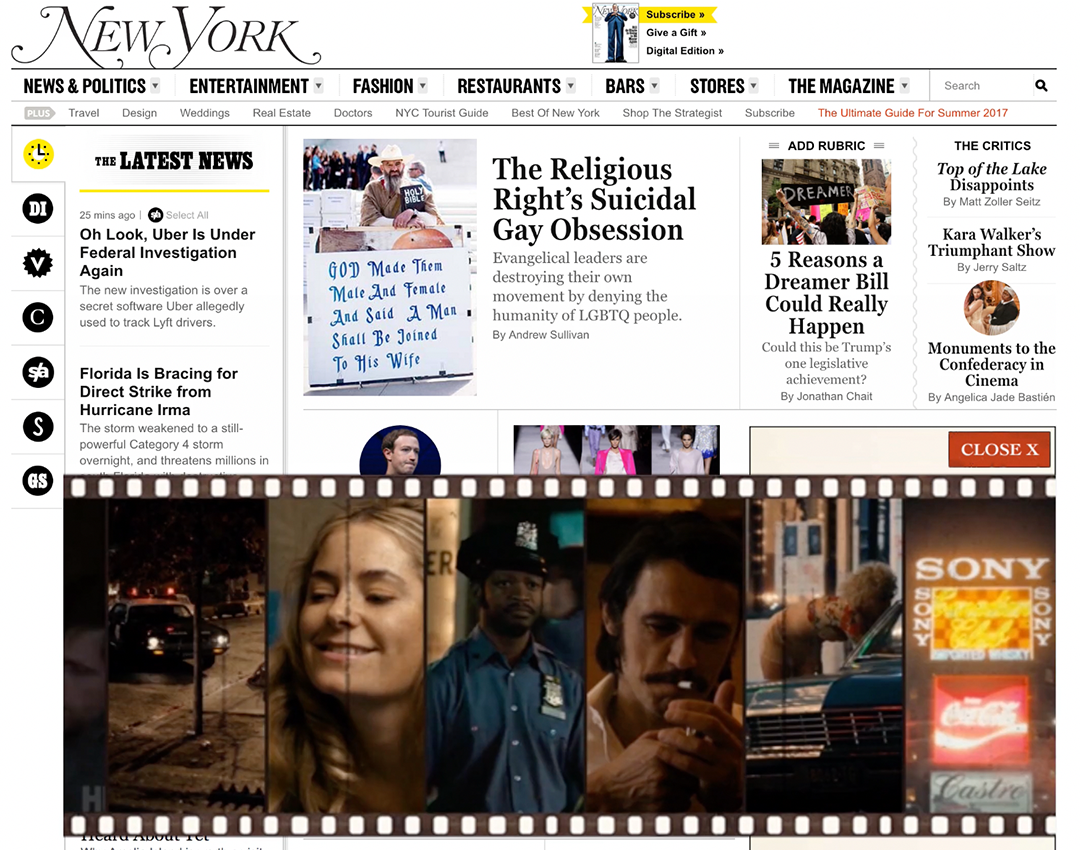A detailed caption for the described image might read:

"A screenshot of the front page from a New York-themed publication, featuring 'New York' prominently in elegant, capital letters at the upper left corner. Adjacent to this title is a large, cartoonish portrait of a man with elongated legs, centered within a black square. To the right of the image is a vertical stack of buttons labeled 'Subscribe,' 'Give a Gift,' and 'Digital Edition.' Below, a black horizontal line stretches across the page, with categories in black capital letters labeled 'News & Politics,' 'Entertainment,' 'Fashion,' 'Restaurants,' 'Bars,' 'Stories,' 'The Magazine,' and a search bar iconified by a magnifying glass.

Further down, more black-capped categories such as 'Travel,' 'Design,' 'Weddings,' 'Real Estate,' 'Doctors,' 'New York City,' 'Tourist Guide,' 'Best of New York,' and 'Shop to Stretch' are listed. In red letters, 'Ultimate Guide for Summer 2017' stands out, flanked by gray text.

On the left sidebar, icons of a clock in yellow and black are seen, followed by 'DIVCSASGS' in monochrome. Under a segment dubbed 'The Latest News,' articles start with a yellow line and continue with brief descriptions. Featured prominently is an image of a man in a hat with a beard, captioned, 'God made them male and female, and said a man shall be joined to his wife,' in blue text. Nearby, an article titled 'The Religious Right's Suicidal Gay Obsession' sits beside a small descriptor.

To the right, a second image depicts protesters with a sign stating, 'Dreamers.' The caption reads, 'Five Reasons Dreamer Bill Could Really Happen,' attributed to Jonathan Chait. Adjacent to this, 'The Critics' features reviews, such as Matt Zoller Seitz's 'Top of the Lake Disappoints' and Jerry Saltz's 'Kara Walker's Triumphant Show,' below which is a small circular icon of two people.

Further below, Angela Jade Ashton's 'Monuments to the Confederacy in Cinema' is mentioned. Cut-off pictures include a known social media mogul and runway models. A filmstrip-like border, both on the top and bottom, showcases scenes of night-time law enforcement interactions, a policewoman, a mustachioed man lighting a cigarette, and a conversation next to a car. Ad slots for Sony, Coca-Cola, and another partially-obscured advertisement are visible, completing the densely-packed overview."